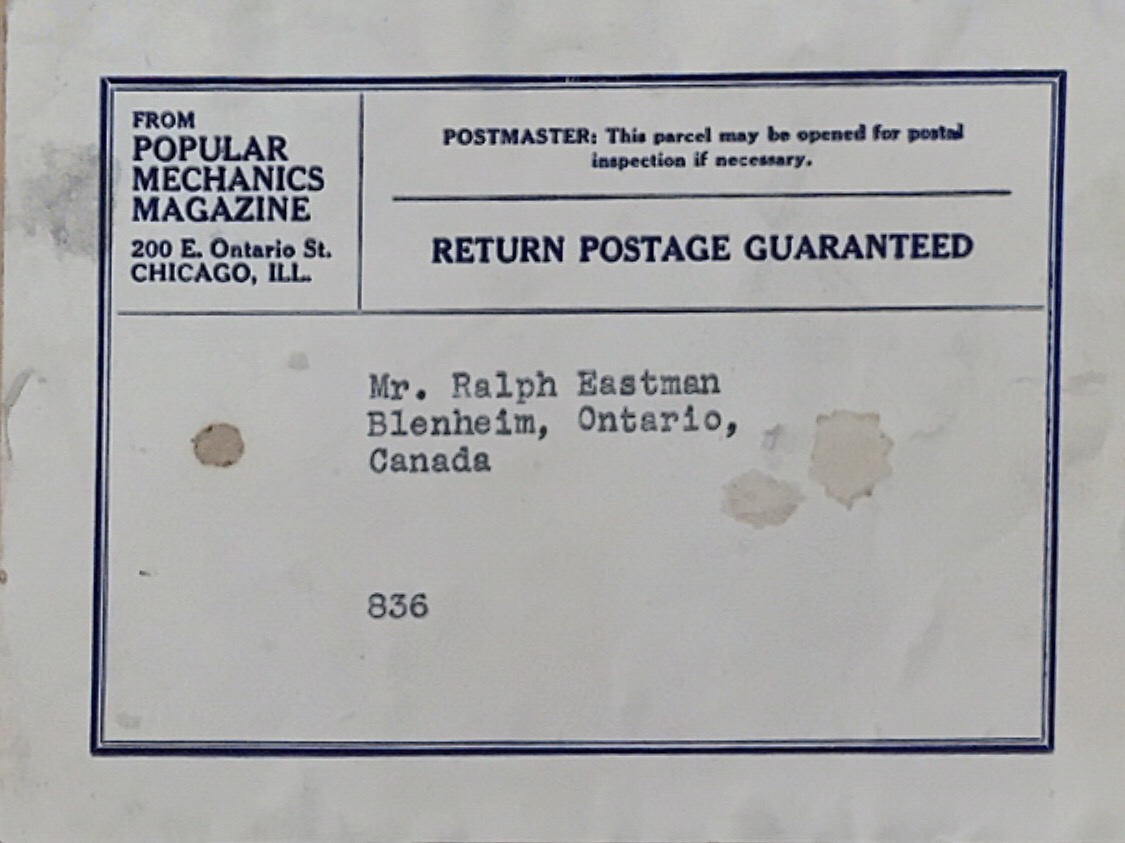This image depicts an aged postal label from a package sent by Popular Mechanics Magazine, located at 200 East Ontario Street, Chicago, Illinois. The label, which is white and encased in a dark blue square frame, bears the address of the recipient, Mr. Ralph Eastman, Blenheim, Ontario, Canada, with the postal code 836, typed clearly at the bottom. At the top of the label, printed in a distinct section marked off in black, are the details "Postmaster, this parcel may be opened for postal inspection if necessary," and "return postage guaranteed." The white background of the label shows signs of aging, with visible watermarks and dirt spots, indicating its well-worn condition.